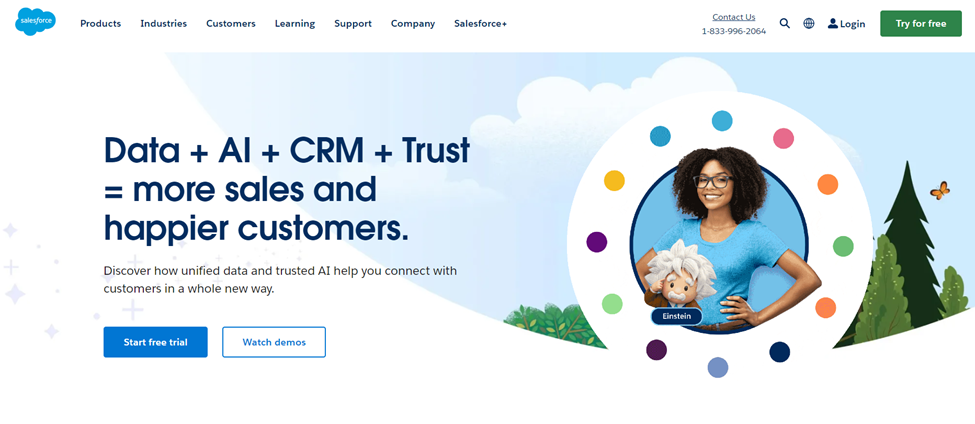The header of the image features a white background with blue text. On the top left, the name "Salesforce" is prominently displayed in white within a blue cloud. Adjacent to this cloud on the right are navigation tabs labeled: Product, Industries, Customers, Lending, Support, Company, and Salesforce Plus. Positioned on the far right is a collection of icons and buttons including "Contact Us" with the number 1-833-996-2064, a search icon, a browser icon, a login icon, and a green button with white text that reads "Try for Free."

The main section of the page features a compelling message on the left side: "Data + AI + CRM + Trust = More Sales and Happier Customers." Below this statement, there's an enticing subtext: “Discover how Unified Data and Trusted AI help you to connect with customers in a whole new way.” Underneath this text are two call-to-action buttons. The first, “Start Free Trial,” is blue with white text, and the second, “Watch Demos,” is white with blue text.

On the right side, there is an image of a woman standing with her hands on her waist, dressed in blue. Next to her, a stylized drawing of Einstein is displayed, labeled "Einstein." The illustration is surrounded by a palette of vibrant colors including blue, pink, yellow, orange, green, maroon, and dark blue. The background is adorned with picturesque green trees and fluffy white clouds, adding a serene and appealing backdrop to the page.